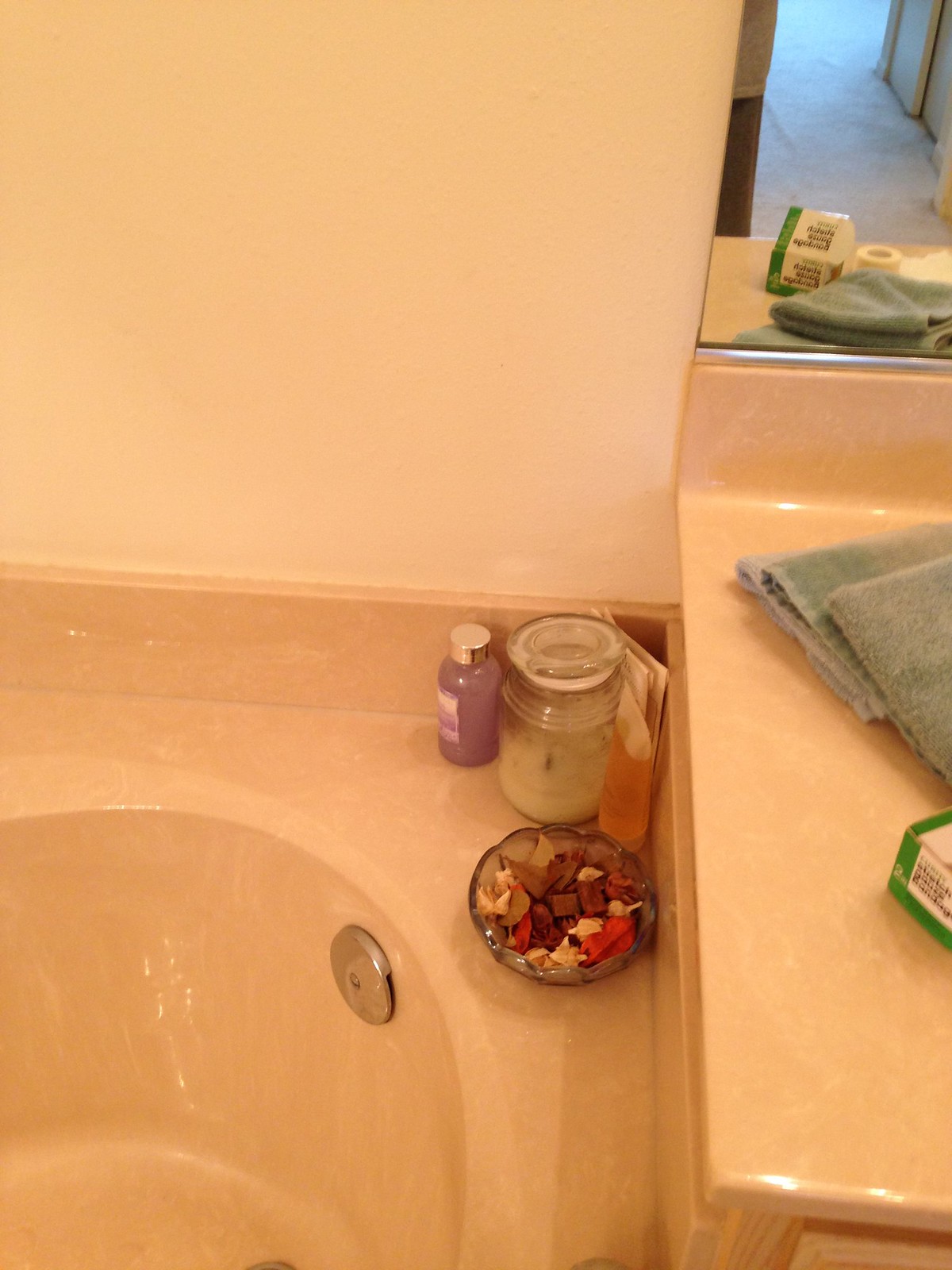This photograph captures a close-up view of a bathroom. In the upper left-hand corner, the cream-colored walls dominate the scene. To the upper right-hand side, a mirror reflects the countertop of the sink in front of it. In the reflection, you can see the light blue carpet flooring, a cardboard box containing gauze tape, and a stack of gray towels. The right side of the image showcases the fiberglass surfaces of the sink and the bathtub, which sit adjacent to each other. The bathtub begins in the bottom left corner of the image, revealing its covered silver drain and deep basin. In the bathtub's corner, various items are arranged, including a candle, a bottle of body lotion, small packets of scented products, and a glass bowl containing colorful pieces of incense.